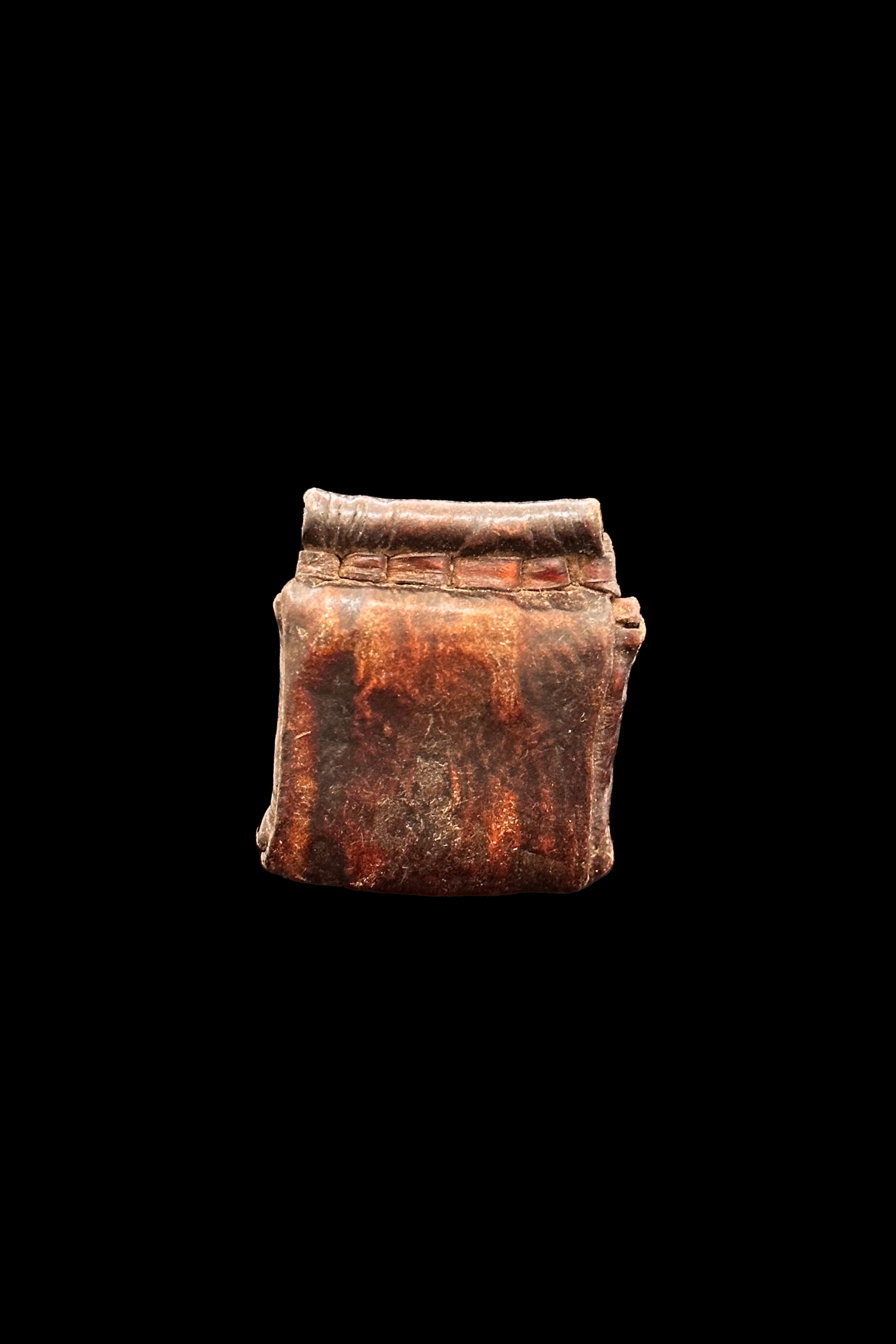This image features an ancient artifact displayed against a completely black background, emphasizing its detailed and intricate design. The central item, rendered predominantly in various shades of brown reminiscent of cooked bacon with darker and lighter patches, appears to be made of an organic material, such as wood or leather. The object has a rolled, curved top leading into several carved or pressed rectangular areas, which continue the curve down to the bottom. The texture and color variations suggest it could be old leather, similar to a well-worn wallet or carrying case, with animal skin features. Additionally, an interesting detail includes an imprint that resembles a Saint Bernard dog's face, lending a unique character to this enigmatic artifact.